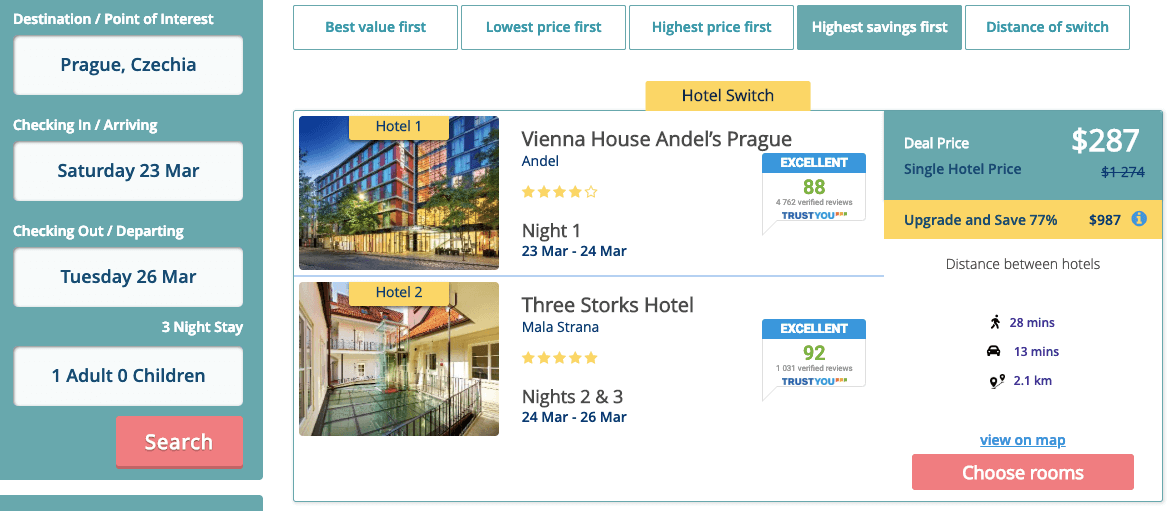A screenshot of a hotel booking website is displayed. On the left-hand side, within a green block, is essential booking information shown in white text. It outlines the destination as Purdue, Czechoslovakia, with a check-in date of Saturday, March 23rd, and a check-out date of Tuesday, March 26th, for a three-night stay. The details specify one adult with no children accompanying the trip. A prominent red "Search" button is located at the bottom right of this menu.

The main webpage features various sorting options at the top, including "Best Value First," "Lowest Price First," "Highest Price First," and "High Savings First," with the latter highlighted in darker green to indicate it is selected. There is also a yellow bar above the main hotel options labeled "Hotels."

The first listed hotel, "Hotel One," includes an image of a large four-story Vienna House hotel. It has a rating of four stars and an "88 Trusted" rating for a stay on the night of March 23rd. The price is highlighted at $287 as the "Deal Price," with a single hotel price of $274 crossed out to indicate a discount.

The second listed hotel, "Hotel Two," presents an image of an indoor scene featuring a middle pool within a three-story hotel, identified as Malastana. This hotel boasts a five-star rating and an "Excellent" rating of 92 for nights two and three, covering March 24th to March 26th. To the right, it notes the distance between hotels as 28 minutes walking, 13 minutes driving, or 2.1 kilometers.

Additionally, users have the option to view the hotels on a map and a red button labeled "Choose Rooms" is available for making a selection.